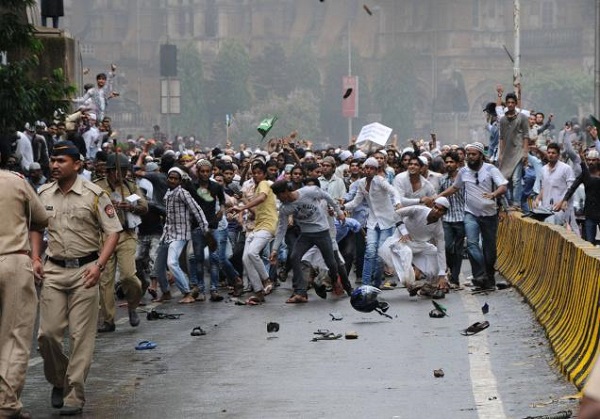This photograph captures a chaotic and escalating riot in India, set on a rain-soaked street. Dominating the scene is a vast and agitated crowd of men, their anger palpable as they surge forward, hurling various objects—including shoes, sandals, and motorcycle helmets—towards the foreground. In the midst of this turmoil, scattered debris litters the ground, evidence of the ongoing unrest. A yellow barricade runs along the right-hand side, delineating the space amid the disorder. On the lower left, three unarmed police officers, dressed in beige uniforms, appear relatively calm and are slowly retreating from the aggressive rioters. Some of the officers lack protective gear, though one at the rear is equipped with a stick and a helmet. The tension between the determined, object-flinging crowd and the stoic, retreating officers underscores the fraught and volatile atmosphere captured in this striking image.